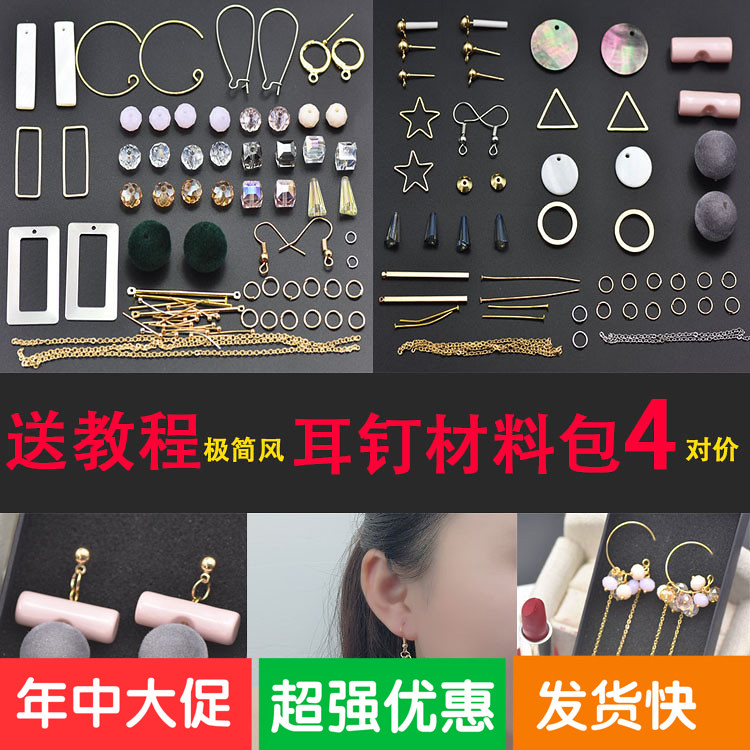This is a detailed image of various types of jewelry, primarily showcasing different styles of earrings, organized into five distinct sections on a slate gray and black background. The top of the image features two larger photos of earrings, including gold hoops, triangular silver earrings, and stud earrings in different designs like pearls and rhinestones. Some earrings are oblong-shaped, while others are star-shaped. In the center, a horizontal banner with foreign writing, possibly in Korean, Japanese, or Chinese, divides the sections. Below the banner are three images; the center one shows a close-up of an ear adorned with an earring, flanked by close-ups of other earrings, including clusters of pearls and gold hoops. Each of these bottom images is framed in colored boxes—red, green, and orange—with white text inside. The bottom also displays a variety of small, tiny hoops and earrings in multiple colors, including white gold, black, gray, pink, and multicolored designs. There's also a glimpse of lipstick at the bottom, adding to the array of accessories.